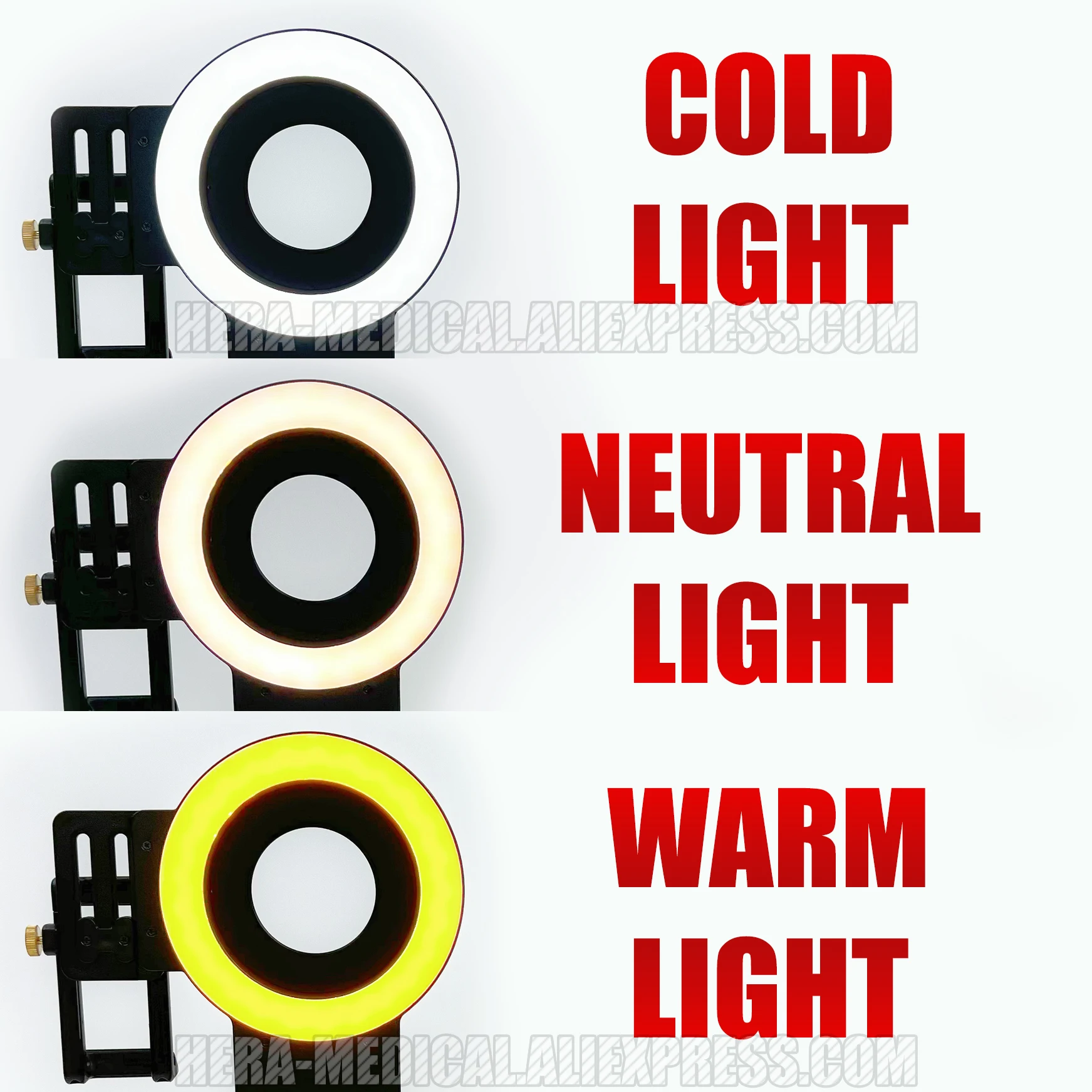This image appears to be a product advertisement from a company selling lighting fixtures, possibly related to medical or stage lighting, as evidenced by the watermark "harrahmedicalalleyexpress.com" visible twice, once at the top and once at the bottom of the image. The advertisement features three vertically aligned circular lights, each mounted with a black circular fixture and supported by what looks like a black rectangular bracket with a securing nut. The lights only vary by the color they emit: the top light labeled "Cold Light" emits a bright white light, the middle light labeled "Neutral Light" emits a pale beige-white light, and the bottom light labeled "Warm Light" emits a bright yellow light. These labels are displayed in bold red text to the right of each corresponding light. The background of the advertisement is white, highlighting the contrast and differences among the three lighting options. The image is detailed and structured to clearly show the varying lighting conditions provided by the fixtures.